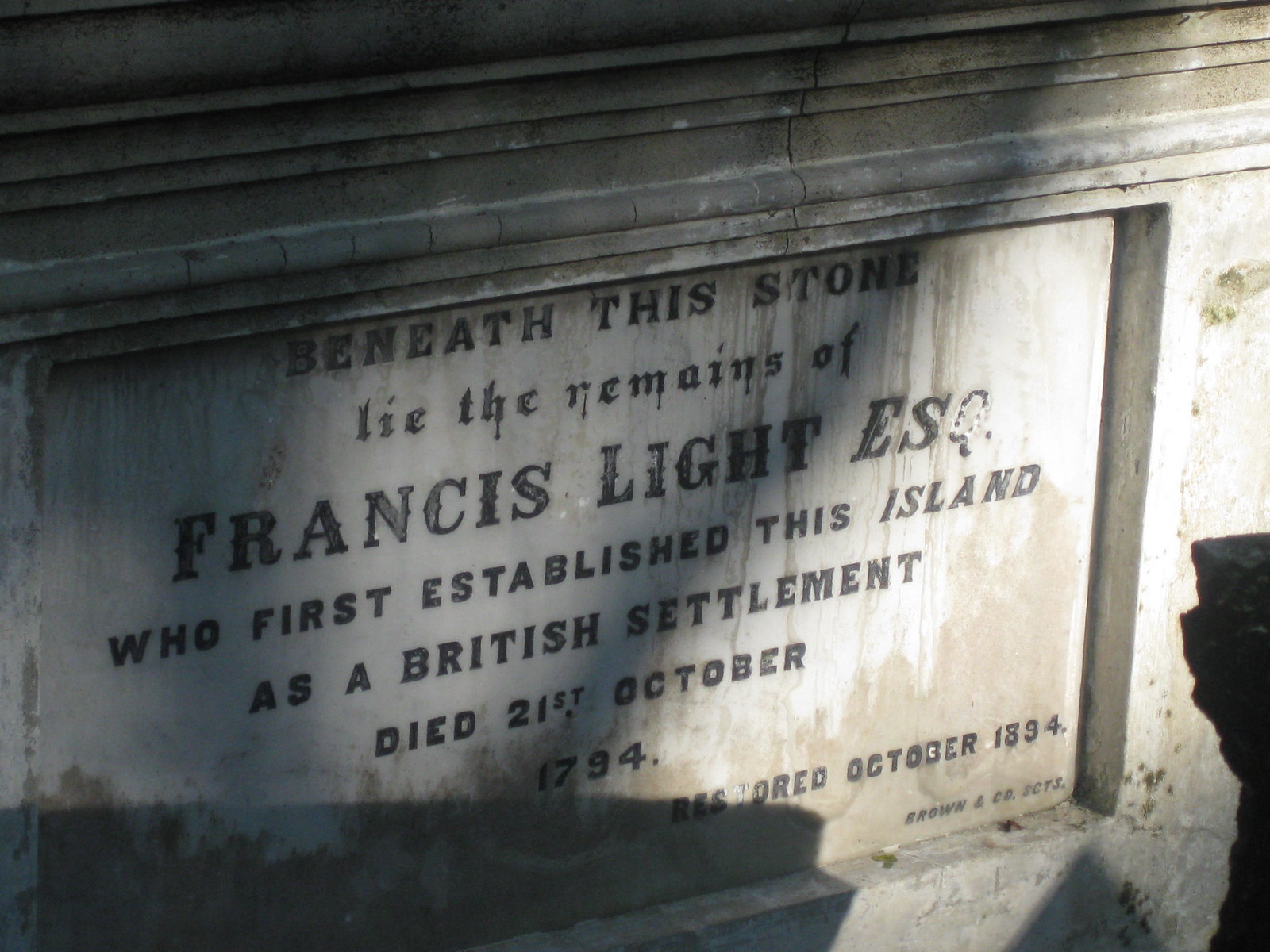The image depicts an old, gray headstone situated in a cemetery, adorned with black engravings that are somewhat worn and weathered. The text on the headstone reads: "Beneath this stone lie the remains of Francis Light, Esq., who first established this island as a British settlement, died 21st October 1794, restored October 1894, Brown and Company." The stone shows signs of age, bearing a few cracks particularly at the top, with noticeable streaks, dirt, and possible mold or mildew, which adds a rugged texture. The headstone is positioned at a slight diagonal in the photograph, with the bottom and middle left being more prominent. A light source illuminates the right side, creating a contrast with the shadowed left side, enhancing the visibility of the stone's details despite its worn condition.